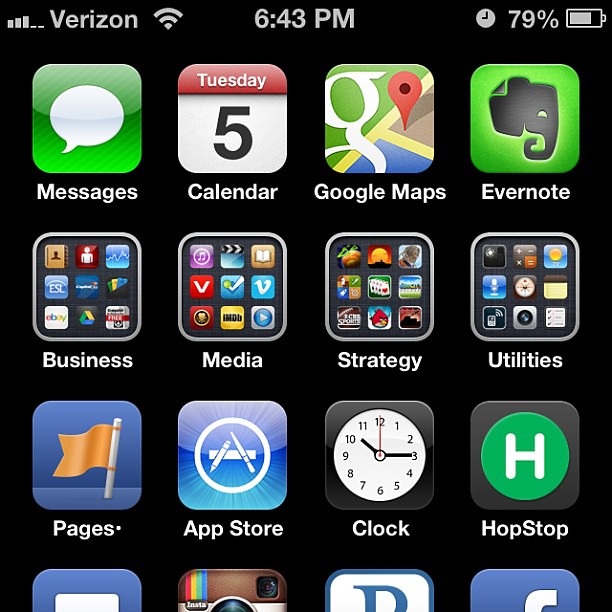A screenshot taken on an iPhone, displaying the home screen against a black background. The status bar at the top shows the Verizon carrier, Wi-Fi signal, three bars of cellular signal, the time as 6:43 PM, and a battery life at 79% with the battery icon nearly full. The alarm symbol indicates that an alarm has been set. The screen date shows it is Tuesday the 5th. Various apps are visible and organized into categorized folders. Notable apps include a calendar, Google Maps, and Evernote, which is identifiable by its green icon featuring an elephant. The "Business" folder contains eBay, ESL, Google, and Contacts apps. The "Media" folder includes IMDb and Venmo. The "Utilities" folder holds clocks, calculators, weather apps, notes, and strategy games. Social media apps like Instagram and Facebook are also present on the screen.